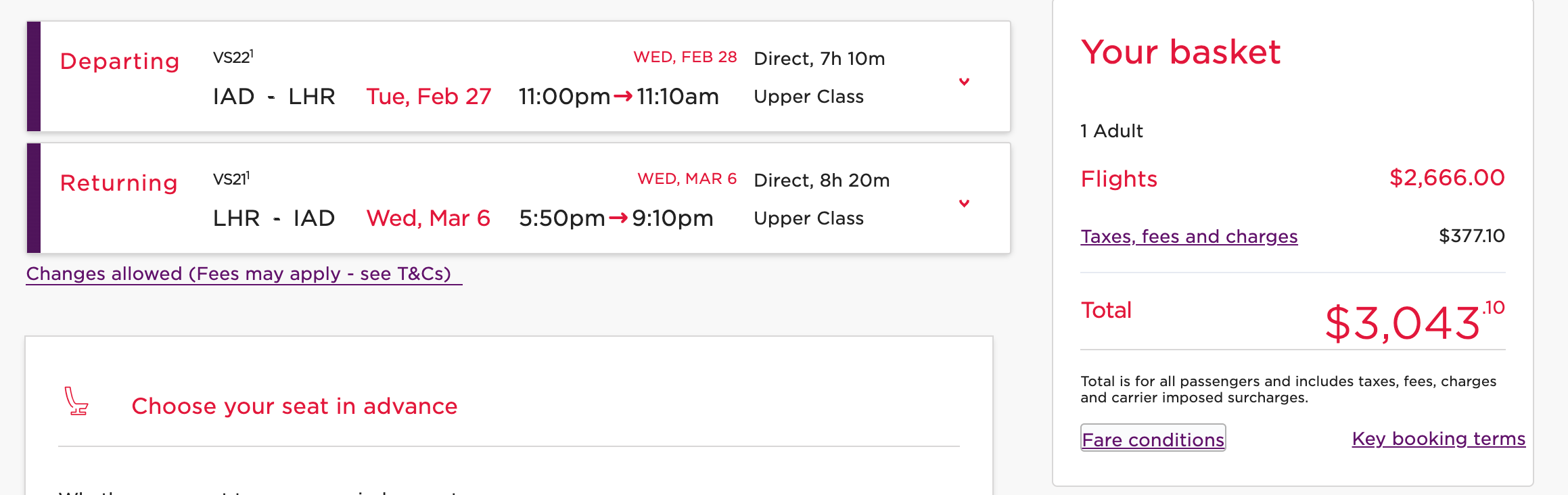This image provides detailed information about a flight booking summary. The entire background has a green tint, while the content is divided into two main sections: the flight details on the left and the pricing on the right.

**Left Side: Flight Details**
- **Flight Information:**
  - There are two white boxes aligned vertically, each with a narrow blue bar on the left edge.
  - **Departure Information:**
    - From: Washington Dulles International Airport (IAD)
    - To: London Heathrow Airport (LHR)
    - Date: Tuesday, February 27
    - Departure Time: 11:00 PM
    - Arrival Time: 10:10 AM (next day)
    - Class: Upper Class
    - Flight Duration: 7 hours and 10 minutes
    - Type: Direct Flight
  - **Return Information:**
    - From: London Heathrow Airport (LHR)
    - To: Washington Dulles International Airport (IAD)
    - Date: Wednesday, March 6
    - Departure Time: 5:50 PM
    - Arrival Time: 9:10 PM
    - Class: Upper Class
    - Flight Duration: 8 hours and 20 minutes
    - Type: Direct Flight

- **Additional Information:**
  - A blue text at the bottom indicates: "Changes allowed, fees may apply. See T's and C's."
  - There’s a button below this section for choosing your seat in advance.

**Right Side: Pricing Details**
- **Your Basket:**
  - Contains a white box with black text summarizing the pricing:
    - One adult's flight: $2,666
    - Taxes, fees, and charges: $377.10
    - Total Cost: $3,043.10

- **Additional Information:**
  - In smaller gray text, there are terms and conditions available underlined in blue, labeled as "fares and conditions and key booking terms."

Overall, the image is a comprehensive display of an airfare booking, highlighting essential flight details and associated costs, with options for further amendments and information.